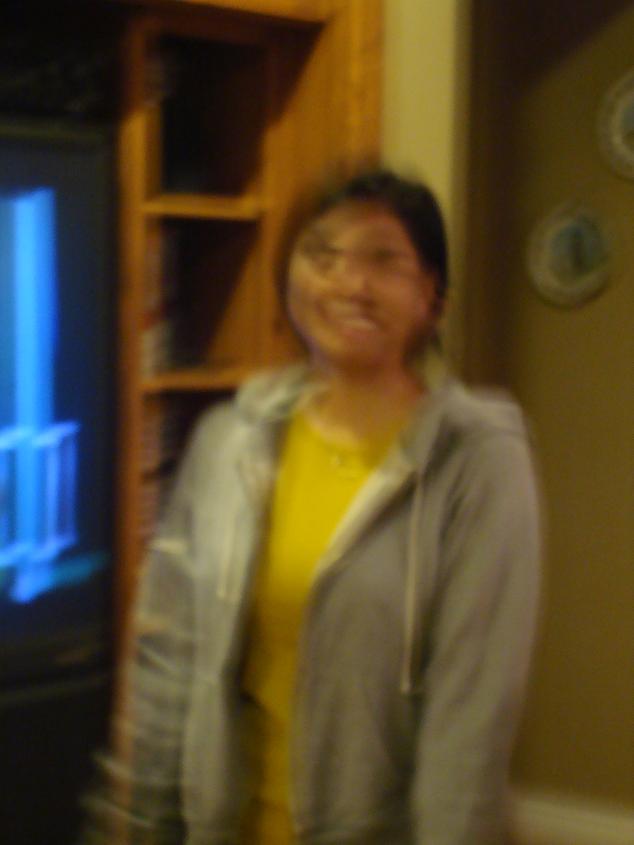This is a very low-quality and blurry photograph reminiscent of an old wind-up camera print. The image, taken indoors under low lighting, appears pixelated and shaky, indicative of the camera moving during the shot. It features a young woman, likely in her late teens or early twenties, standing in the center. She has short black hair and is wearing glasses. She is dressed in a grey hoodie with a hood that has pull ties, which is unzipped to reveal a yellowish, possibly lime green shirt beneath. The woman is smiling, despite the overall distortion. In the background, one can discern elements that suggest an indoor setting, possibly on a ship due to the presence of round porthole-like windows, but it is equally plausible to be a room with items such as a ladder, a bookcase, and a turned-on TV. There’s also mention of a fluorescent neon bluish light and a hallway with beige walls adorned with decorative china plates.